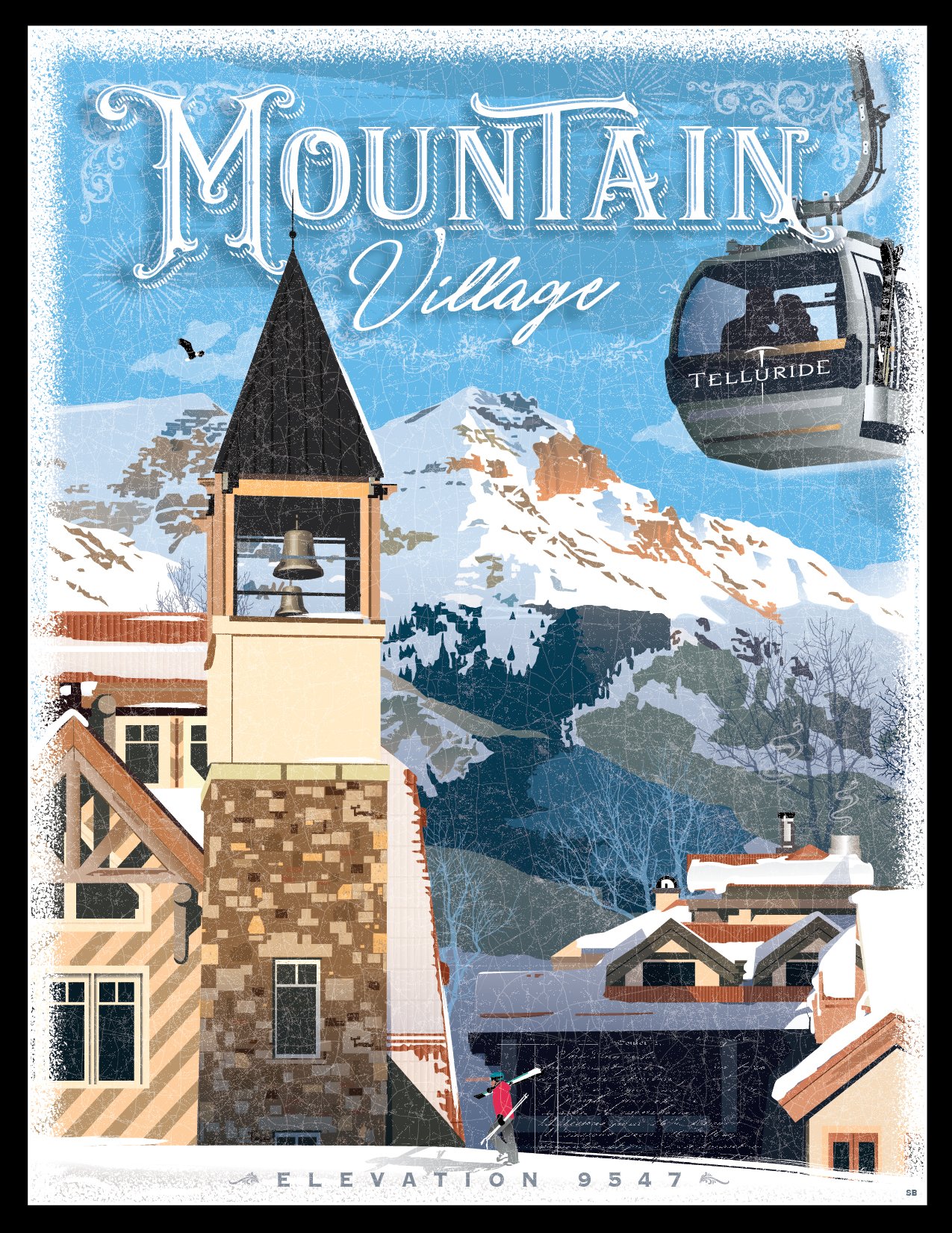The image is a detailed poster advertising "Mountain Village" at Telluride. Dominating the scene is a majestic, snow-covered mountain in the background, casting a shadow over the picturesque resort. In the top left corner, the text "Mountain Village" stands out, with "MOUNTAIN" in all capital white letters and "village" in cursive.

A small, snow-dusted church with a prominent black steeple, housing two visible bells, is positioned in the bottom left. Nearby, several buildings also sport snowy roofs, enhancing the quaint village atmosphere. On the right side of the image, a gondola ski lift, marked with "Telluride" and carrying two men and a woman, ascends, illustrating the resort’s skiing allure. 

A solitary skier in a red jacket can be seen in the middle of the scene, navigating the snow-covered paths below the text. Above it all, a bird, possibly an eagle, soars freely in the sky. The elevation of 9,547 feet is clearly stated at the bottom, emphasizing the high-altitude charm of the resort. The entire poster is encased in a black frame, adding a polished touch to the advertisement.